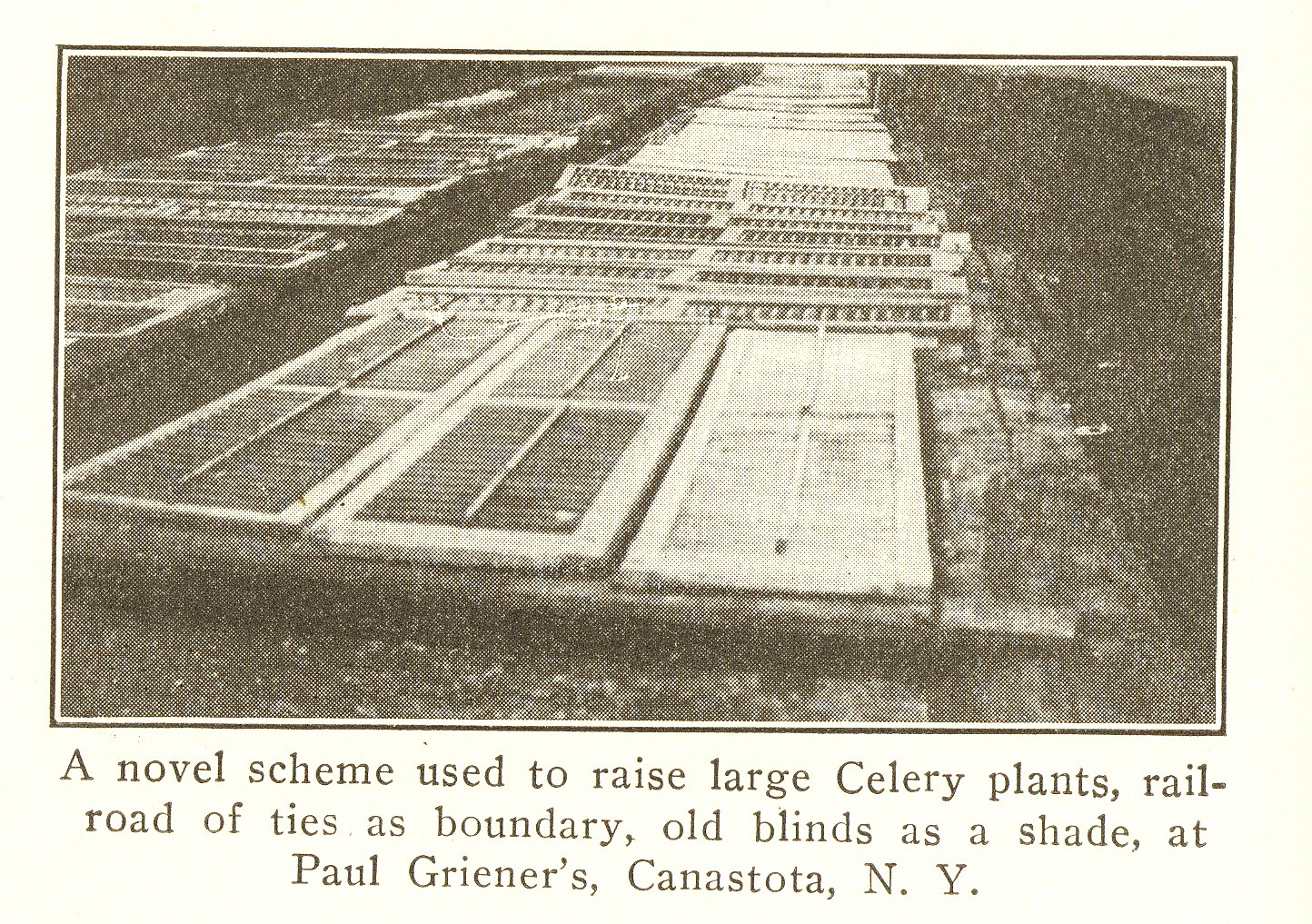This aged and sepia-toned black-and-white photograph, likely sourced from an old newspaper, portrays a makeshift agricultural setup at Paul Greiner's in Canastota, New York. The image, surrounded by a distinct black border, features rows of window blinds or panels arranged horizontally, alongside what appear to be railroad ties used as boundaries. The grainy and faded quality of the picture gives it an antique, almost historical charm. Beneath the photograph, a caption reads: "A novel scheme used to raise large celery plants. Railroad of ties as boundary, old blinds as a shade, at Paul Greiner’s, Canastota, N.Y." The overall effect is reminiscent of a bygone era, capturing an innovative, large-scale outdoor greenhouse setup.